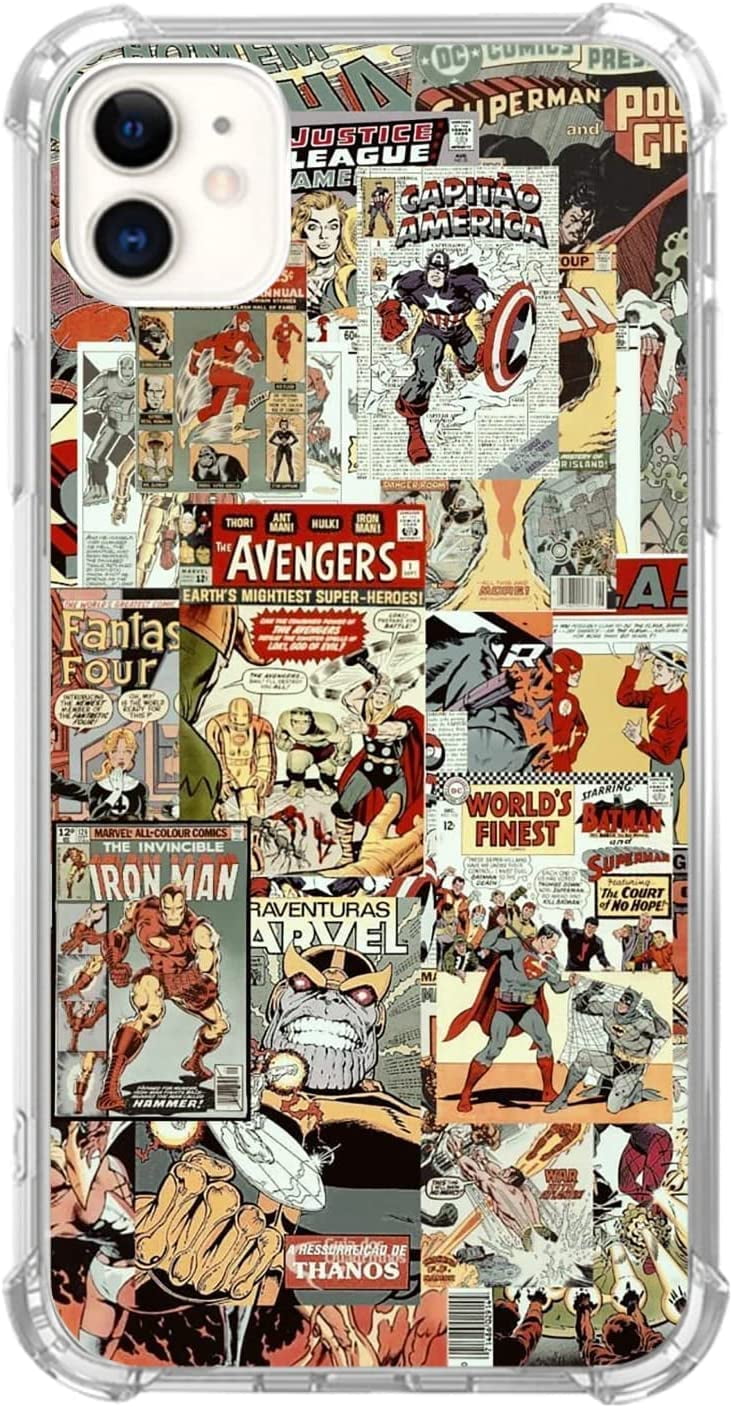This image showcases the back of a modern smartphone encased in a clear protector with edges that highlight its dual camera lenses in the upper left-hand corner. The phone case is adorned with a collection of vintage comic book images, giving it an aged appearance. The decorative comic book covers feature superheroes and notable characters from both Marvel and DC universes, including titles such as The Avengers, Iron Man, Captain America, the Justice League, Superman, Thanos, and the Fantastic Four. The color palette is rich yet muted, dominated by hues of olive, gray, white, dark red, black, and shades of brown and yellow, adding to the nostalgic feel. Scattered across the case are miniature scenes and iconic figures, from alien landscapes and spaceships to barcodes and comic strips, capturing the essence of classic comic book artistry.